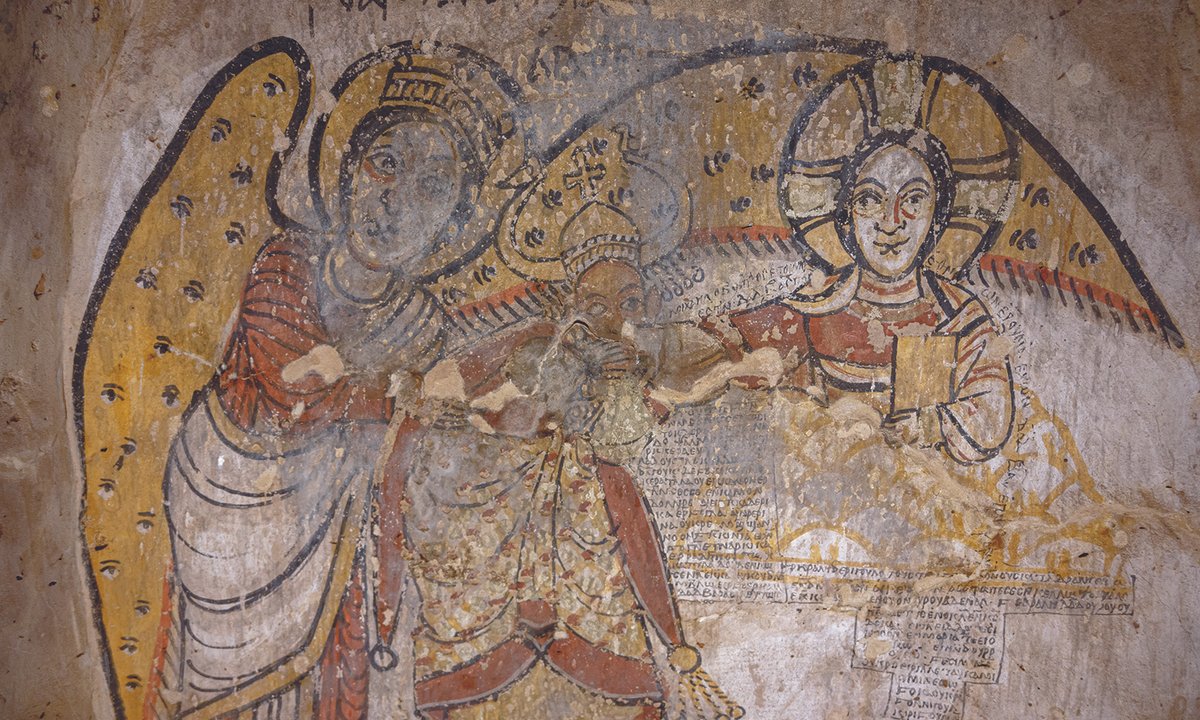This image depicts an ancient, faded painting on a light brown stone wall, likely in an old building and possibly of biblical significance. The composition features three figures. On the left, an angel with large, yellow wings speckled with black and bordered in black, wears a long robe—white on the bottom and red on top—and has a yellow head covering with arches resembling a halo. In the center stands a figure, possibly an ecclesiastical figure, adorned with a yellow cap featuring a cross and a robe with red and yellow tassels. The figure to the right wears a form-fitting yellow headpiece like an Egyptian headdress and a yellow gown. Intricate but smudged details obscure some parts of the painting, and there is illegible text beneath the third figure, possibly in Greek.